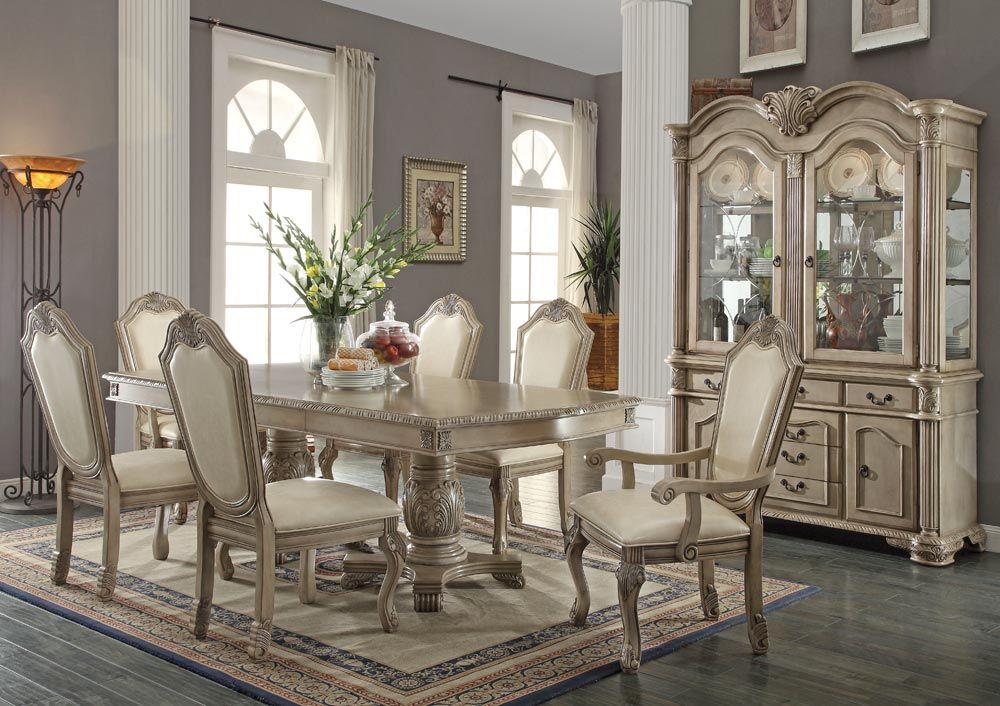The image depicts a modern dining room with gray walls and two white-pillared windows framed by white curtains. The room features a large white wooden dining table that seats six, with one chair pulled out, inviting one to sit. Each chair has a wooden frame with white leather cushions. The floor is a stylish gray wood, partially covered by a rug with a white, blue, and red border under the table. To the right, a china cabinet made from the same material as the table holds silverware and other items behind glass doors. The table is adorned with vibrant decor, including a vase of yellow and white flowers and a jar of apples. A lighting sconce hangs above, and a picture of flowers is displayed between the windows, enhancing the room's welcoming, homey atmosphere.